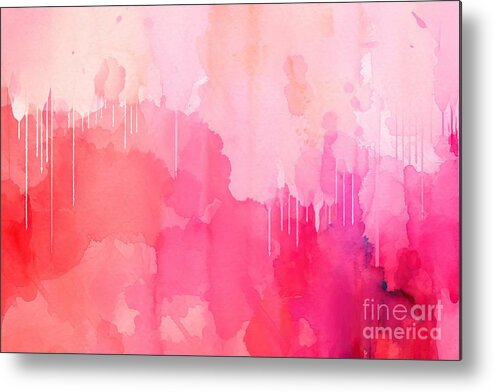This rectangular abstract painting, appearing slightly tilted with shadows cast along the bottom and right-hand side, seems to be either hung on a wall or presented against a white background. Encased in an ultra-thin black frame, the artwork prominently features varying shades of pinks and reds, with the colors transitioning from darker tones at the bottom to lighter, almost white hues at the top. The painting resembles a wash of watercolors with splotches and blobs blending seamlessly together, creating an ethereal effect. Thin white lines appear where the light pinks meet the darker pinks, dripping in straight lines of various lengths, concentrated at the center. The bottom right corner bears a faint watermark reading "Fine Art America" in lowercase white letters, adding a subtle mark to this soft, yet dynamic piece of art.